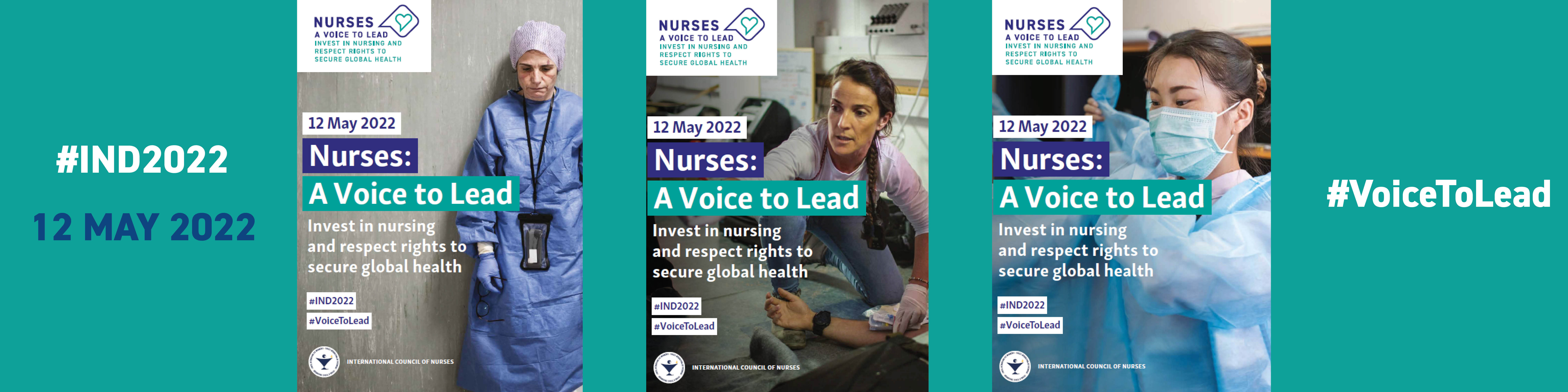The image consists of a horizontal rectangle with a teal green background, divided into three sections by three vertical rectangular posters aligned side by side. Each poster carries a theme centered around nurses and their importance. 

On the left side of the background, in bold text, is the hashtag "IND 2022". Below that, the date "12th of May 2022" denotes an important event. On the far right of the background, another hashtag reads "Voice to Lead".

Each of the three central posters features different images of nurses but shares similar textual content. Prominently displayed is the phrase, "12th of May 2022, Nurses: A Voice to Lead," followed by the slogans, "Invest in Nursing" and "Respect Rights to Secure Global Health". 

In the top left corner of each poster, the phrase "Nurses: A Voice to Lead" is inscribed, although a portion of the text remains too small to decipher. The overall design aims to emphasize the key message of honoring and investing in nursing to advance global health.